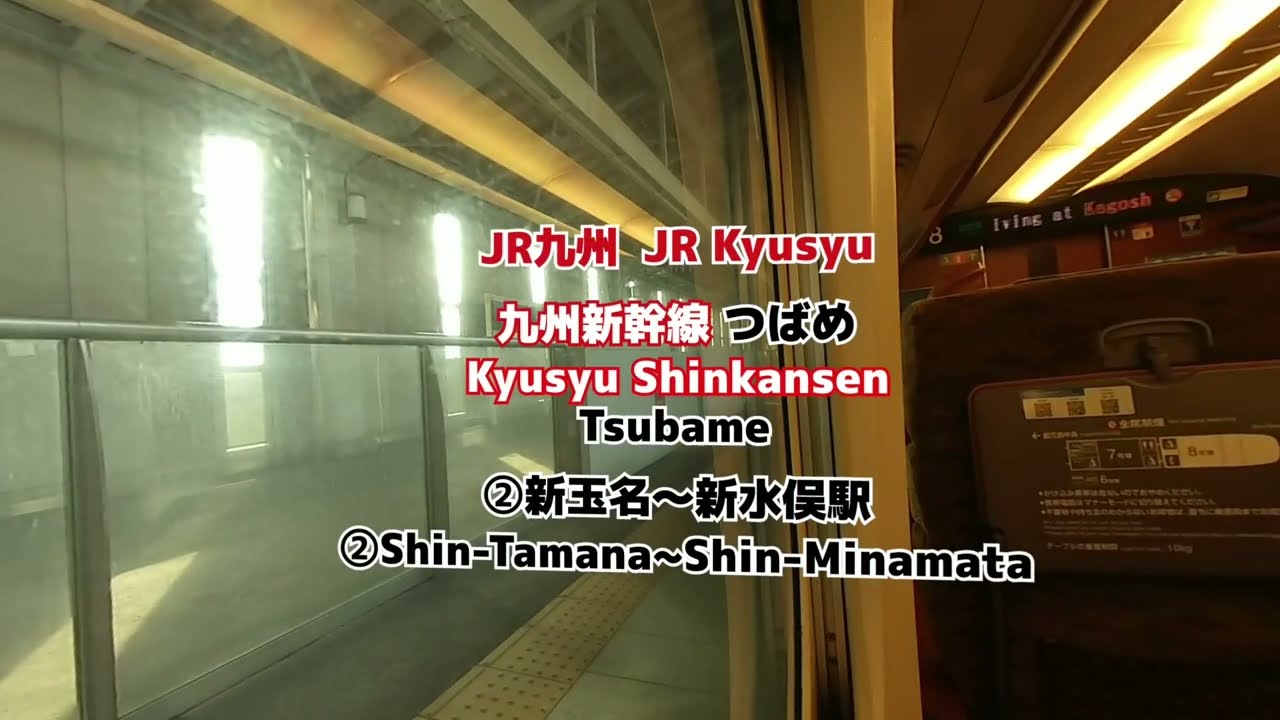The image portrays the indoor setting of a Japanese train or train platform, identified by both Japanese and English text indicating names like "JR Kyushu," "Shin-Tamana," and "Shin-Minamata." On the left-hand side, there's a series of plexiglass windows extending diagonally from the lower left to the upper right. Adjacent to this, a gray walkway stretches alongside a divider wall. To the right of this divider wall, there appears to be a section resembling the back of a train seat, complete with a tray table setup and a rectangular halogen light above. Centered in the image, various pieces of signage and branding are visible in both Asian characters and English, highlighted in red and black writing. The area is well-lit, with yellow-tinted lights overhead, contributing to the industrial, yet orderly atmosphere.